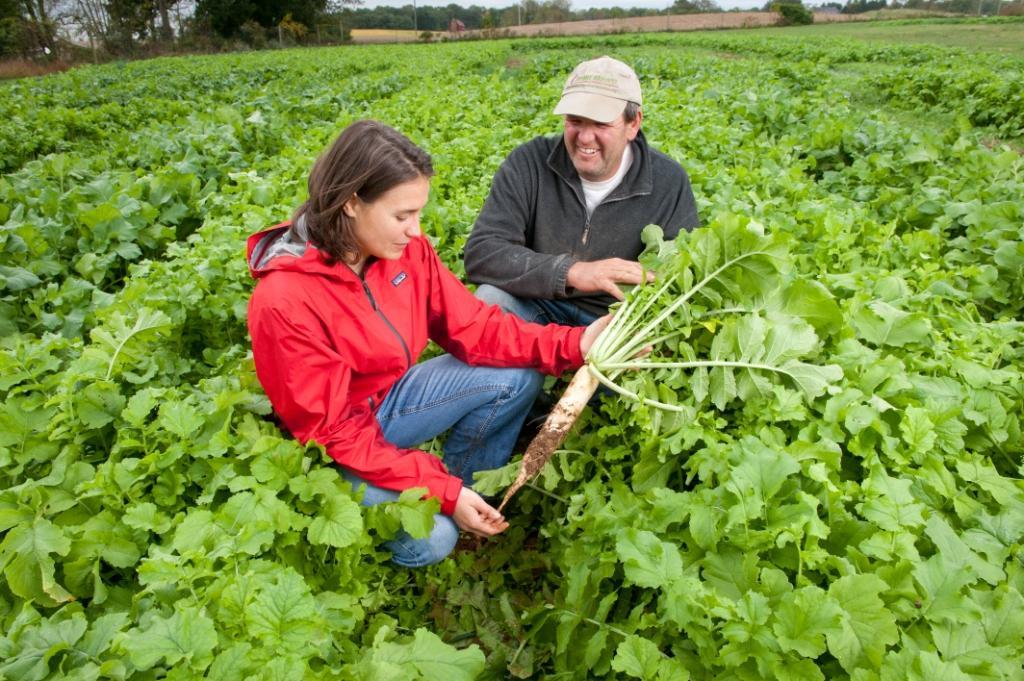In this image, you see a vibrant farmland blanketed in lush green leafy plants that stretch out as far as the eye can see. The scene is bathed in sunlight, adding a warm and cheerful ambiance. Centrally featured in the image are two individuals, a woman and a man, both kneeling amidst the thriving crops.

The woman, positioned on the left, has shoulder-length straight brown hair and is wearing a bright red hooded Patagonia zip-up jacket paired with jeans. She is intently examining a large, dirt-covered parsnip that she has presumably just pulled from the soil. The parsnip is held primarily in her left hand, with her right hand offering additional support. Her gaze is fixed on the impressive vegetable, showcasing a moment of connection with her harvest.

Next to her, the man, who is slightly older, is also kneeling. He sports a beige cap and a charcoal gray three-quarter zip-up sweater, complemented by jeans. His expression is one of amusement and pride, as he looks towards the woman and the parsnip she holds. They both share a moment of joy and accomplishment in this bountiful, leafy field.